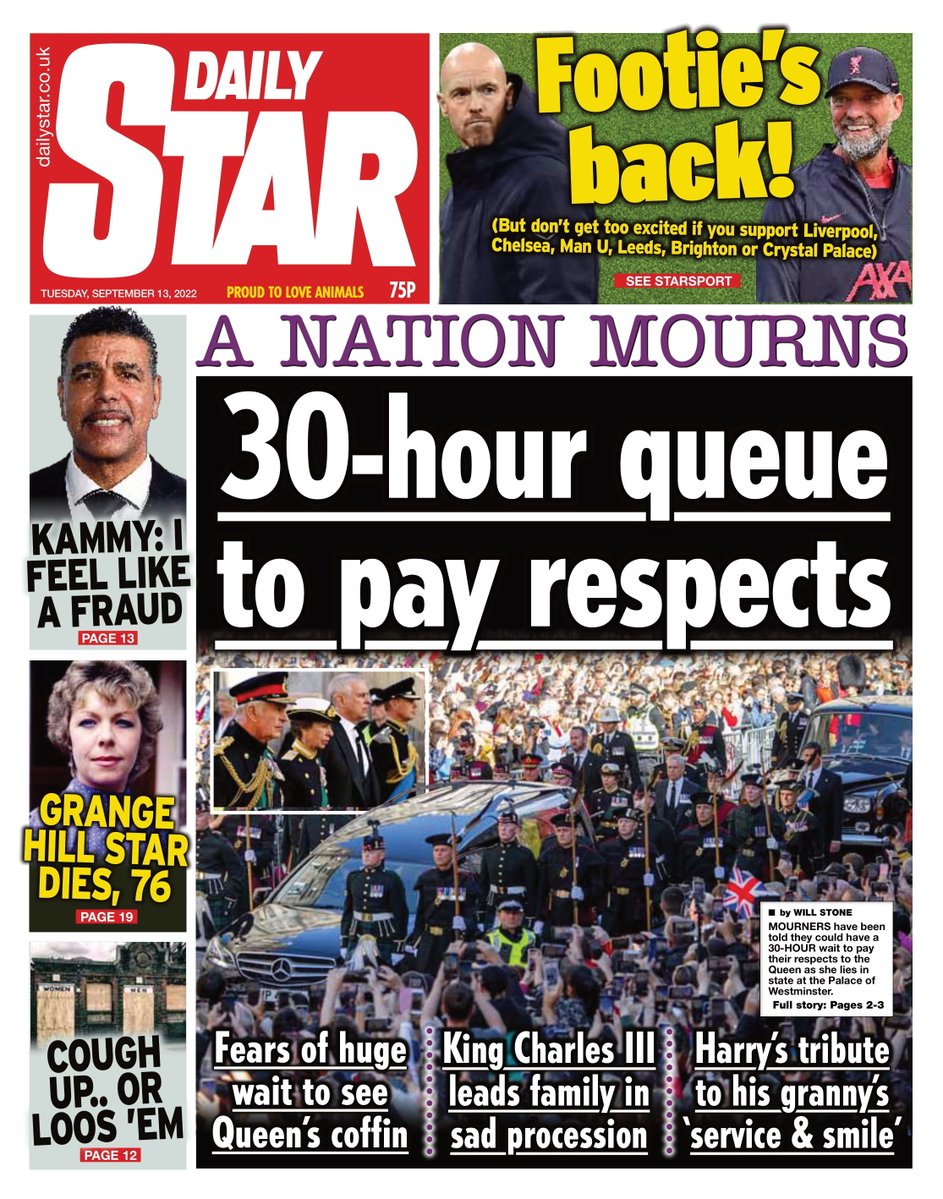In this image, we see a screenshot of the front cover of the Daily Star publication. The upper left corner features a red box with large, bold, white text that reads "Daily Star", along with the website URL "dailystar.co.uk" displayed just above it. Directly below this is the publication date in small white text, "Tuesday, September 13, 2022."

Moving to the right, the most eye-catching element is the headline in bright yellow block print, stating: "Footie's back, but don't get too excited if you support Liverpool, Chelsea, Man U, Leeds, Brighton or Crystal Palace." 
  
Below the bold headline are images of two men: on the right, a man with a gray beard and mustache, wearing a baseball cap; and on the left, a bald man dressed in a dark jacket.

Just beneath these images, another headline is framed within a white banner with the text "A Nation Mourns." Underneath this, on a black background, white bold text announces: "30-hour queue to pay respects."